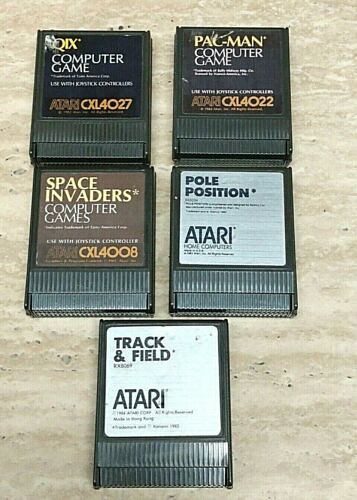A collection of five vintage Atari cartridge-style video games displayed on a tan, porous surface resembling a countertop. The cartridges are rectangular and vertically oriented, akin to the size of a floppy disk. Arranged in a distinctive layout, a single cartridge rests at the bottom, with four others positioned in two rows of two above it. The bottom cartridge features the game "Track & Field" by Atari, identifiable by its silver label. In the middle row, the left cartridge is "Pole Position" by Atari Home Computers, also sporting a silver label. Adjacent to it on the right is "Space Invaders" by Atari, marked with a brown label and coded CXL4008. In the upper row on the left is "QIX," labeled as Atari CXL4027, and to its right is "Pac-Man," coded Atari CXL4022.